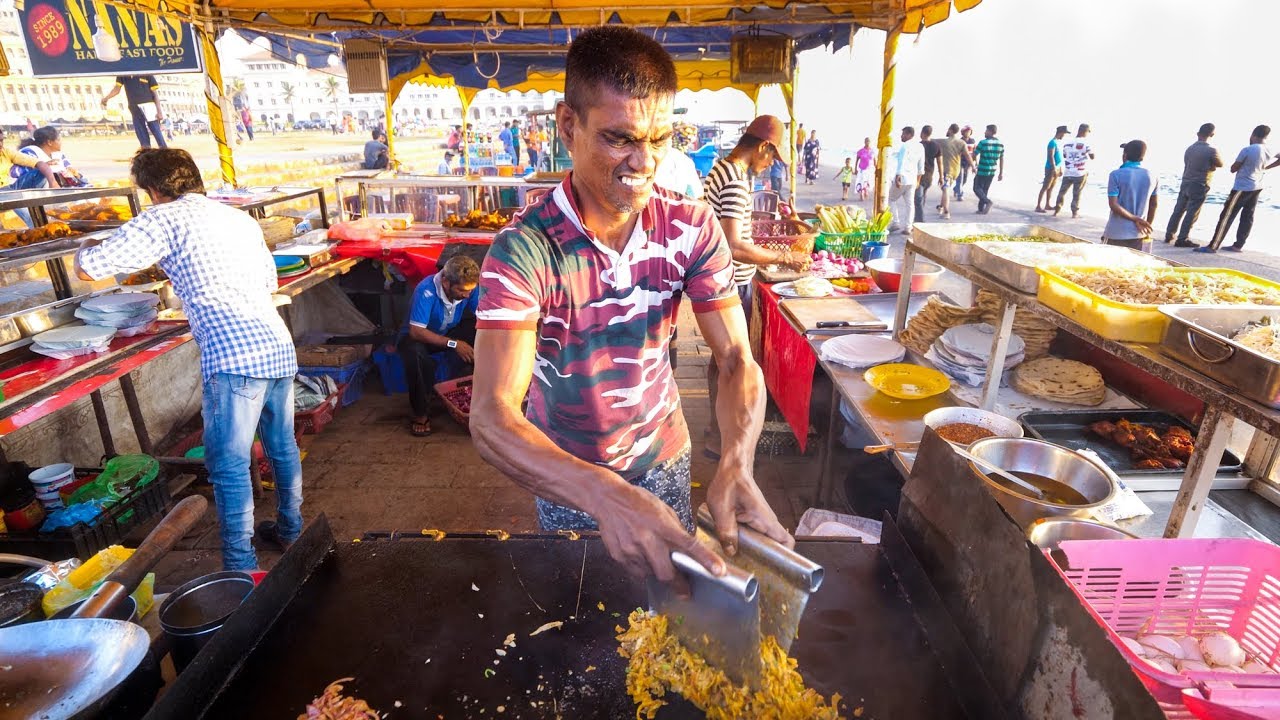In the foreground of this vibrant, full-color photograph taken during a bright, sunlit day, a man is deeply focused on his task at an outdoor street food booth near a beach. He energetically chops up what appears to be chicken on a flat-top grill using two yellow spatulas. His brow is furrowed and he squints, possibly from the intensity of the sun. He sports a camouflage-patterned polo shirt in red, white, and black. 

Surrounding him, the lively scene includes other workers, one in a checkered shirt, busily preparing meals, contributing to the bustling ambiance. In the background, tall white buildings, likely hotels, line the horizon, establishing the setting as a beachside sidewalk cafe. People mill about the area, some potentially customers, enhancing the festive environment. On the left side and further back, more booths and activities are visible, indicating a lively street food market atmosphere by the beach.